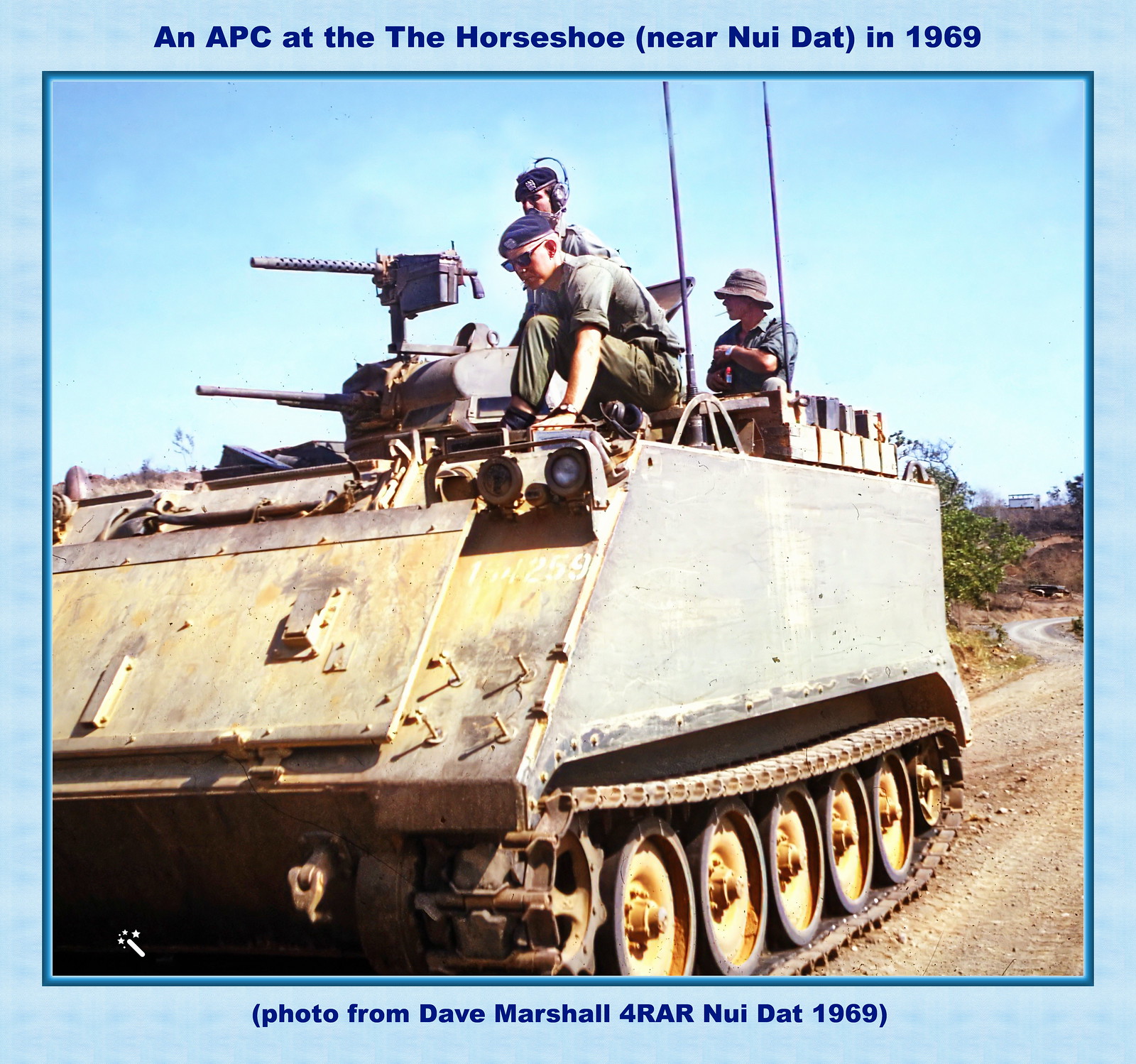The color photograph captures a modern tank moving along a dirt road under a clear blue sky. Atop the tank, which is covered in brown and yellowish dirt and dust, sit three soldiers dressed in army-style uniforms. The soldier in the front sports sunglasses and a beret, the middle one wears a beret with headphones, and the one at the back dons a bucket hat. The scenic background features green trees and foliage, suggesting a survey or preparation activity. The picture is framed with a dark teal border and a light blue outer border. In dark blue lettering above the image, it reads "An APC at the Horseshoe near New Dot in 1969." Beneath the image, it is captioned "Photo from Dave Marshall for RAR New Dot 1969."